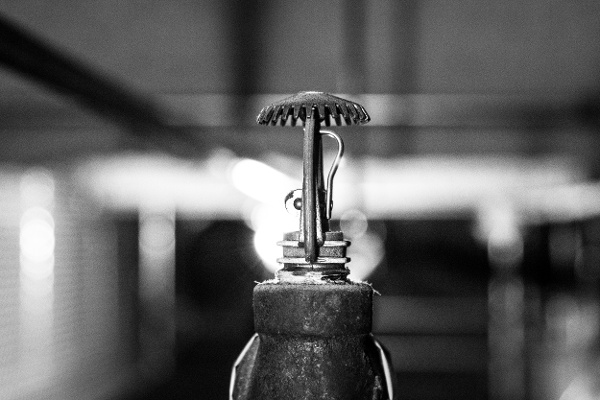In this black and white close-up image, the focus shifts to a mysterious, metallic object prominently situated in the lower middle of the frame. The object resembles a serrated mushroom or umbrella cap, with jagged edges creating a distinctive top. Descending from this cap are two parallel metal bars that connect to a cylindrical base, which appears to be either metal or stone. Extending outward from the cylindrical base is another metal bar branching out perpendicularly to the right and curving downward.

On the left side of the base, there is a noticeable circular wheel, which features a smaller inner wheel at its center. Below this assembly, there are two stacks of horizontal bars. The background is a blurred expanse of gray, punctuated by a horizontal metal bar stretching from the center towards the upper left corner and intersected by vertical beams on both sides. The background gives off an impression of blurry lights and indistinct objects, adding to the enigmatic atmosphere of the photograph.